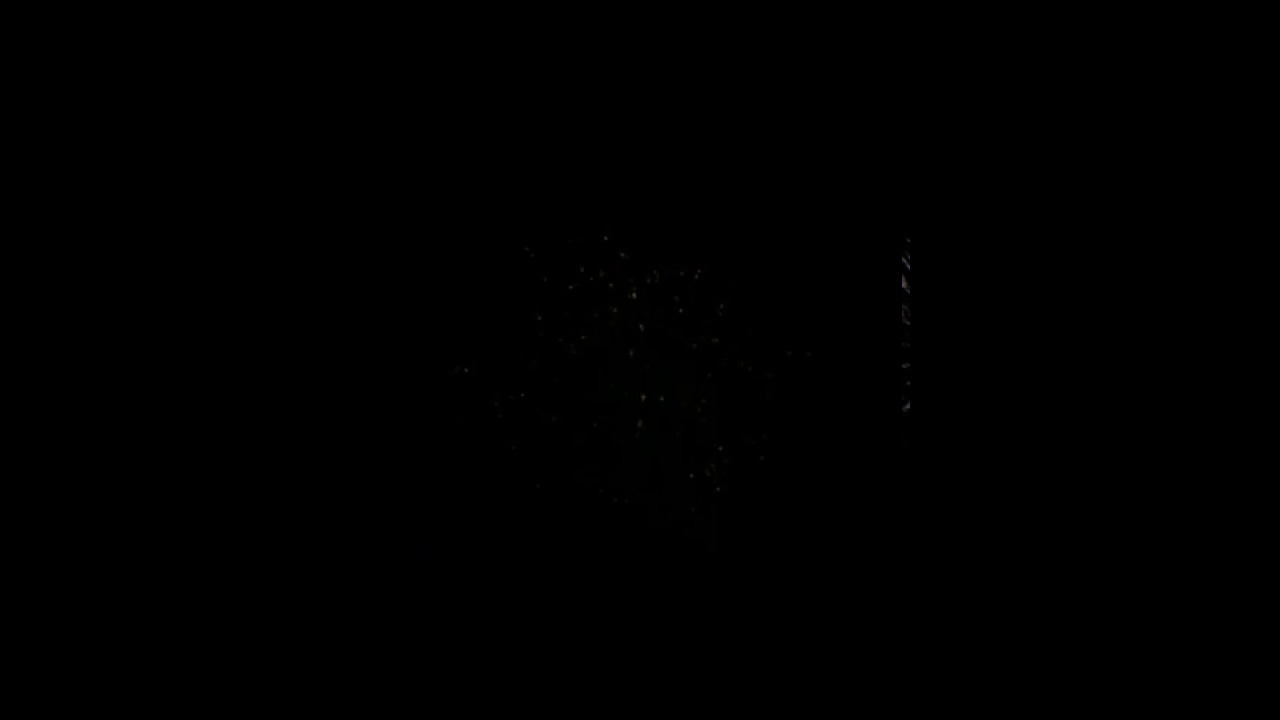The image is a horizontally aligned, landscape-oriented black rectangle with no text or visible images except for subtle details in the center and to the right. At the center, there are faint gray or white specks, resembling dim lights or stars in a dark sky, creating a slightly blurred effect. To the right of these scattered dots, there's an inconsistent, light gray line, appearing as a series of faded slats or segments. The rest of the image is uniformly solid black, providing a stark contrast to the faint details at the center and right side.